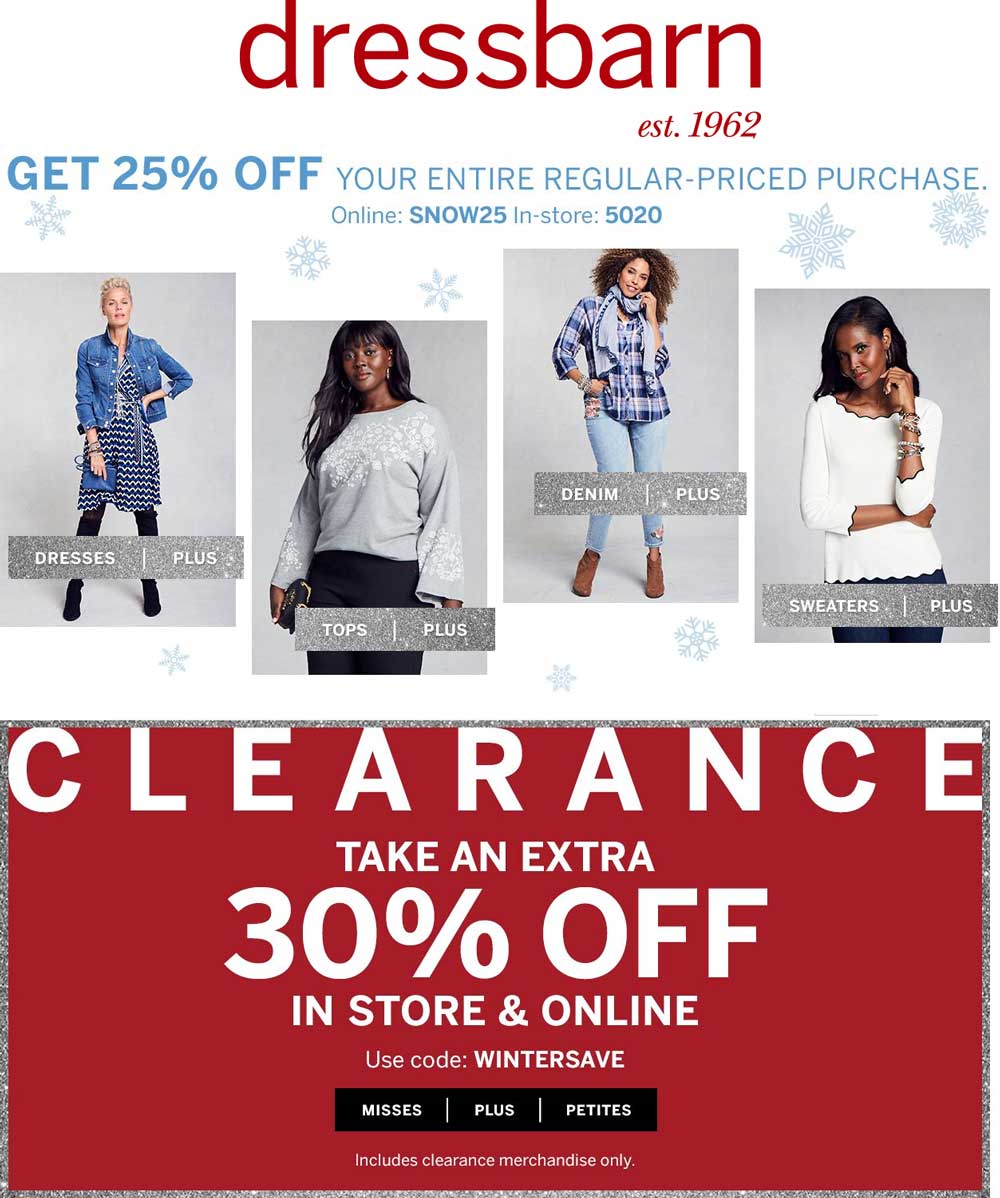**Dress Barn Advertisement**

- **Header**: 
  - **White Background**
  - **Red Text**: "dressbarn" (all lowercase)
  - **Blue Text**: "EST. 1962 Established in 1962"

- **Promotion**:
  - **Large Blue Font**: "GET 25% OFF" (bold)
  - **Regular Font in All Caps**: "YOUR ENTIRE REGULAR-PRICE PURCHASE"
  
  - **Online Code**:
    - **Bolded Text**: "SNOW25"

  - **In-Store Code**:
    - **Bolded Text**: "5020"

- **Design Elements**:
  - **Background**: Snowflakes
  - **Product Images**:
    - **Image 1**: 
      - **Light-skinned Woman**: 
        - **Outfit**: Denim jacket, black and white patterned dress, black knee-high boots
        - **Accessory**: Blue clutch
        - **Label**: "DRESSES + " (white text on silver, sparkly background)
        
    - **Image 2**: 
      - **Dark-skinned Woman**: 
        - **Outfit**: Gray/silver sweater with snowflake design, dark pants
        - **Accessory**: Clutch
        - **Label**: "TOPS + " (white text on sparkly gray/silver background)
        
    - **Image 3**:
      - **Person of Color**:
        - **Outfit**: Blue scarf with dark blue fringe, long sleeve flannel shirt, ripped jeans
        - **Accessory**: Bracelets
        - **Footwear**: Brown boots
        - **Label**: "JEANS + " (white text on sparkly background)

    - **Image 4**:
      - **Dark-skinned Woman**:
        - **Outfit**: White scalloped sweater (3/4 sleeves), dark pants
        - **Label**: "SWEATERS + " (white text on sparkly silver background)

- **Clearance Section**:
  - **Banner**:
    - **Text**: 
      - **Top**: "CLEARANCE" (all caps)
      - **Middle**: "Take an extra 30% OFF" (large letters)
      - **Bottom**: "In-store & Online" 
      - **Code**: "WINTERSAVE" (all caps)
      - **Note**: Text reads "Misses + Petite, includes clearance merchandise only," on a red background.